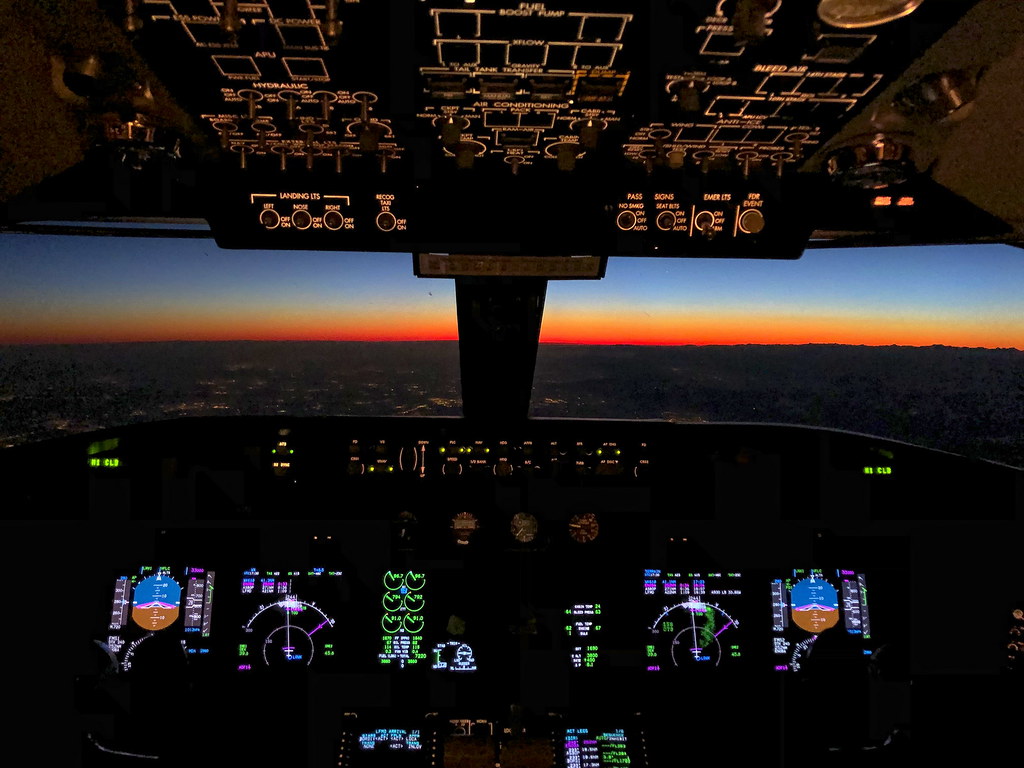This photograph captures the interior view of an airplane cockpit in flight during either the twilight hours of sunset or just before sunrise. The cockpit, likely from a newer large aircraft, is equipped with an array of digitized screens and illuminated control buttons. At the top of the cockpit, a panel of knobs, dials, and control modules is visible, while a secondary array of controls, along with multiple colorful LCD screens, occupies the lower section. These screens display essential flight information such as radar data, elevation, and weather conditions, and are lit up in vibrant neon shades of green, purple, orange, and blue.

Through the clear cockpit window, the scene beyond is mesmerizing. The horizon gradually transitions from a glowing red and orange near the ground to a yellow hue, finally blending into a deep blue sky. The ground below is shrouded in darkness, making it difficult to discern specific details of the cityscape except for the scattered amber lights of buildings and streets, which faintly outline the urban landscape. The airplane is likely at cruising altitude, flying steadily, with no airports visible in the dim expanse below.